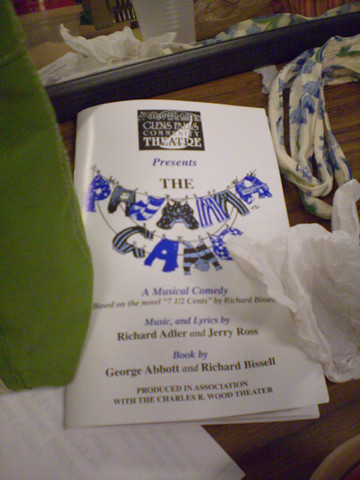This color photograph captures a theater program cover for the play "The Pajama Game." The program, printed on glossy white paper, features text in blue, white, and green. At the top, there is a square box with theater information and a spotlight effect behind the type. Below this, the word "presents" appears, followed by "The Pajama Game," where the letters are creatively formed from images of pajamas and other clothing items such as sweaters and pants, arranged to represent each letter. Striped pants shape the 'M' and a curled sweater forms the 'A,' designed in a playful mix of black, blue, and white. Further down, it mentions it is 'A Musical Comedy' with music and lyrics by Richard Adler and Jerry Ross, and the book by George Abbott and Richard Bissell, produced in association with Charles R. Wood Theater. The program is landscape-oriented and appears to be casually placed on a table amidst various clutter, including a piece of green sweater, a tissue, a cup, and other scattered items. The overall scene provides a realistic, slightly chaotic backdrop to the otherwise neatly designed program.